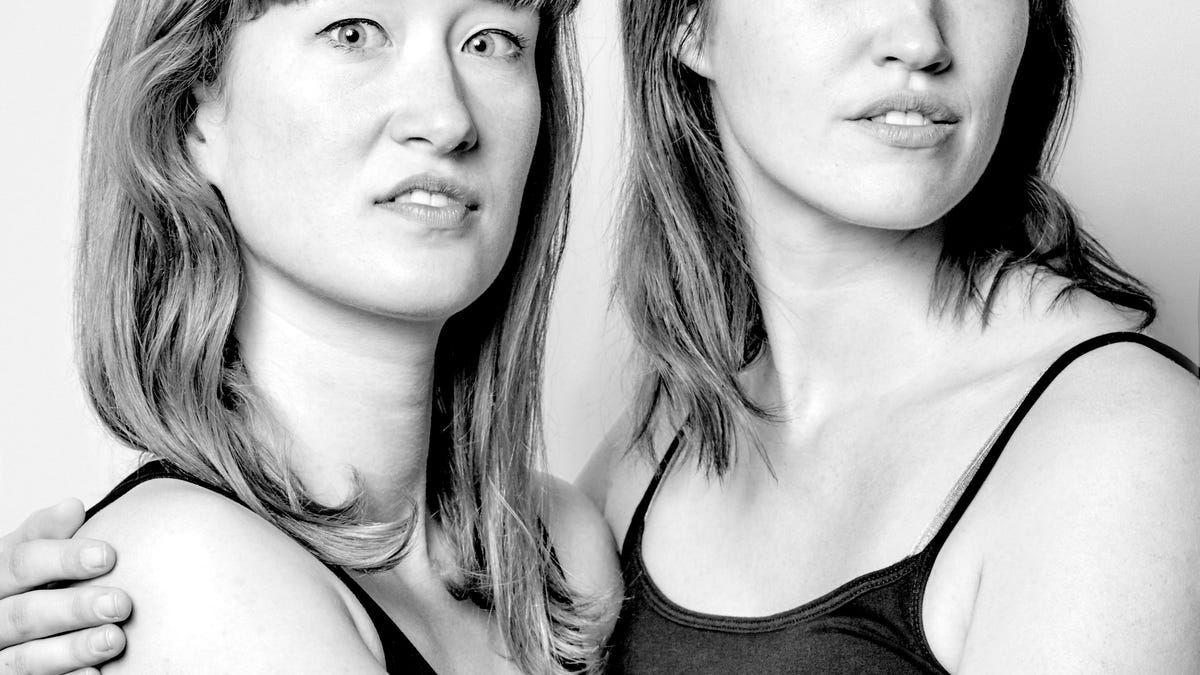In this striking black-and-white photograph, two Caucasian women are captured from just below their shoulders up. The woman on the left, who appears slightly shorter, gazes wide-eyed at the camera as if surprised or shocked. She has straight, light-colored hair that drapes just below her shoulders and wears a black string tank top. Meanwhile, the taller woman on the right, whose face is partially cut off with only her nose and lips visible, also sports straight, light-colored hair that reaches her shoulders. She, too, dons a similar black sleeveless tank top. Both women give a soft, almost hesitant smile, adding an air of subtle mystery to this clean and well-composed image.